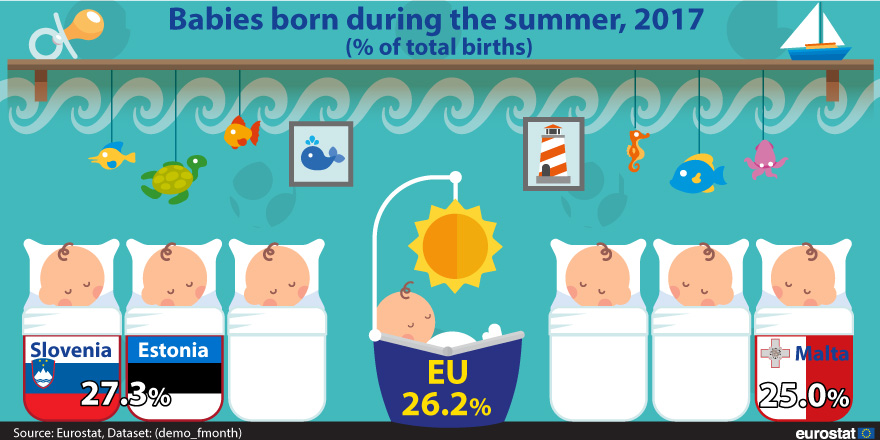The image is a digitally created scene with a baby blue background. At the top center, in darker blue font, it reads "Babies Born During the Summer, 2017" with "(Percent of Total Births)" written underneath in parentheses. The left and right sides feature baby pacifiers with blue handles and yellow nipples, along with white and blue toy sailboats.

A wooden shelf is depicted, and the wall below showcases lighter shades portraying waves, sea turtles, fish, whale illustrations, and a white house. The lower section of the image has babies sleeping in white cribs.

On the left-hand side, the flags of Slovenia (white, blue, and red) and Estonia (blue, black, and white) are displayed, each with the text "27.3%" in white, indicating the percentage of total births for those countries. Adjacent to the flags is a baby without any accompanying text.

At the center, a large blue bassinet with a sun hanging above it holds a sleeping baby. Inside the bassinet, in yellow text, it says "EU 26.2%."

To the right, there are two white bassinets, and next to them is the flag of Malta (white and red). Above this flag, the text "25%" in white indicates Malta's percentage of total births.